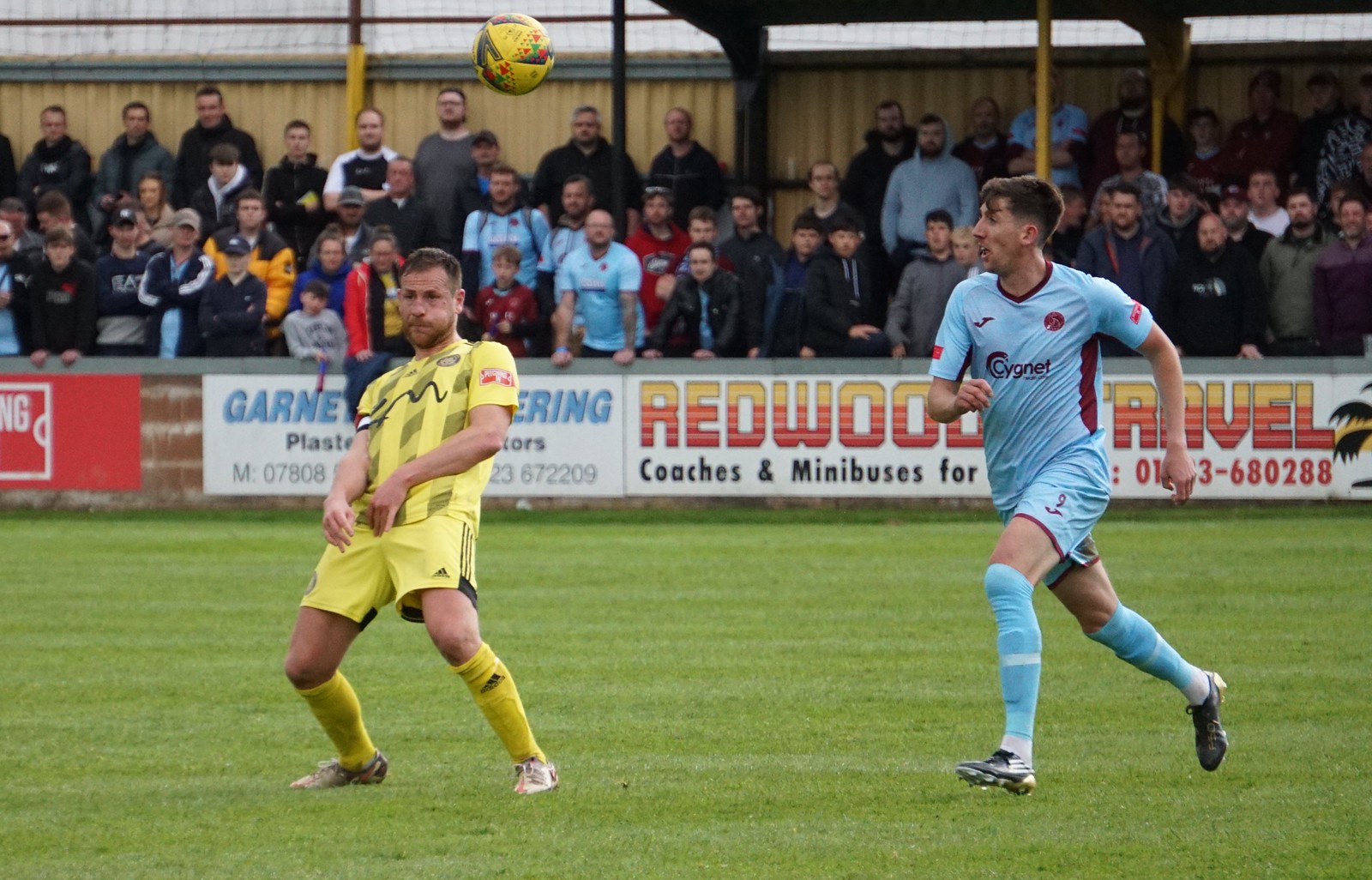The image captures an intense moment in a soccer game on a lush green field. Two male players, both Caucasian, are sprinting towards the action. The player on the left is dressed in a complete yellow soccer uniform, from his jersey and shorts to his socks, and he appears to be focused on a yellow and black soccer ball suspended in mid-air, likely after just making contact with it. The player on the right is clad in a light blue and black jersey, blue shorts, and blue socks, as he charges towards his opponent. Behind the field, a fence and barricades with various company logos such as "Redwood Travel" serve as a boundary. An audience stands behind these barricades, watching intently. Some of the displayed advertisements in the background are "Garnett Learning" and "Coaches and Minibuses" alongside the contact information "013-680288". The image vividly depicts not only the live action on the field but also captures the vibrant atmosphere of the spectators.